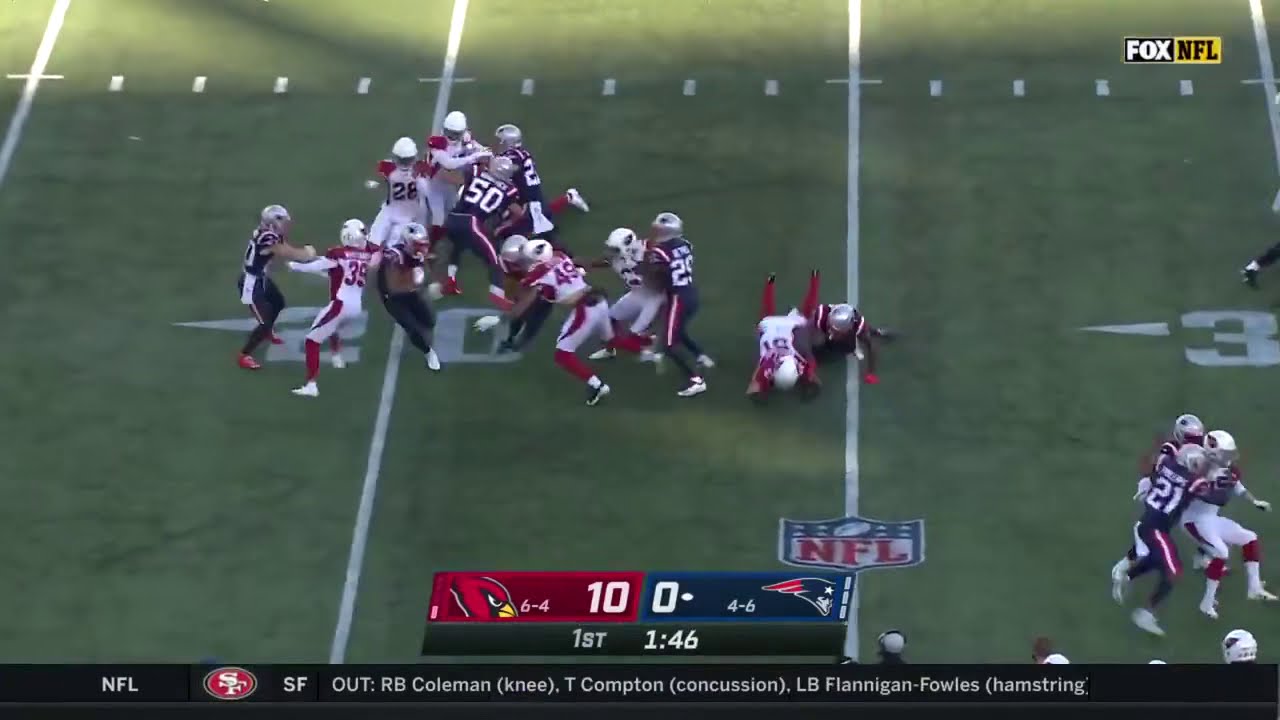This detailed image captures a broadcast screenshot of an NFL football game between the Arizona Cardinals and the New England Patriots. The scene is set on the green field marked with yard lines, prominently showing the 20-yard line where a group of players are tackling each other. The Cardinals, in red and white uniforms with white helmets, are playing against the Patriots, dressed in dark blue and white uniforms with silver helmets. The score displayed at the bottom shows the Cardinals leading with 10 points against the Patriots' 0, with a notation indicating it's the 1st quarter with 1:46 remaining. The image also features the Fox NFL logo in the upper right corner and a black stripe at the bottom with white text reading, "NFL," followed by injury updates: "SF out: RB Coleman (knee), T. Compton (concussion), LB Flanagan (hamstring)." The overall composition of colors and uniforms, alongside the myriad of details and symbols, suggests a typical broadcast presentation on Fox NFL TV.